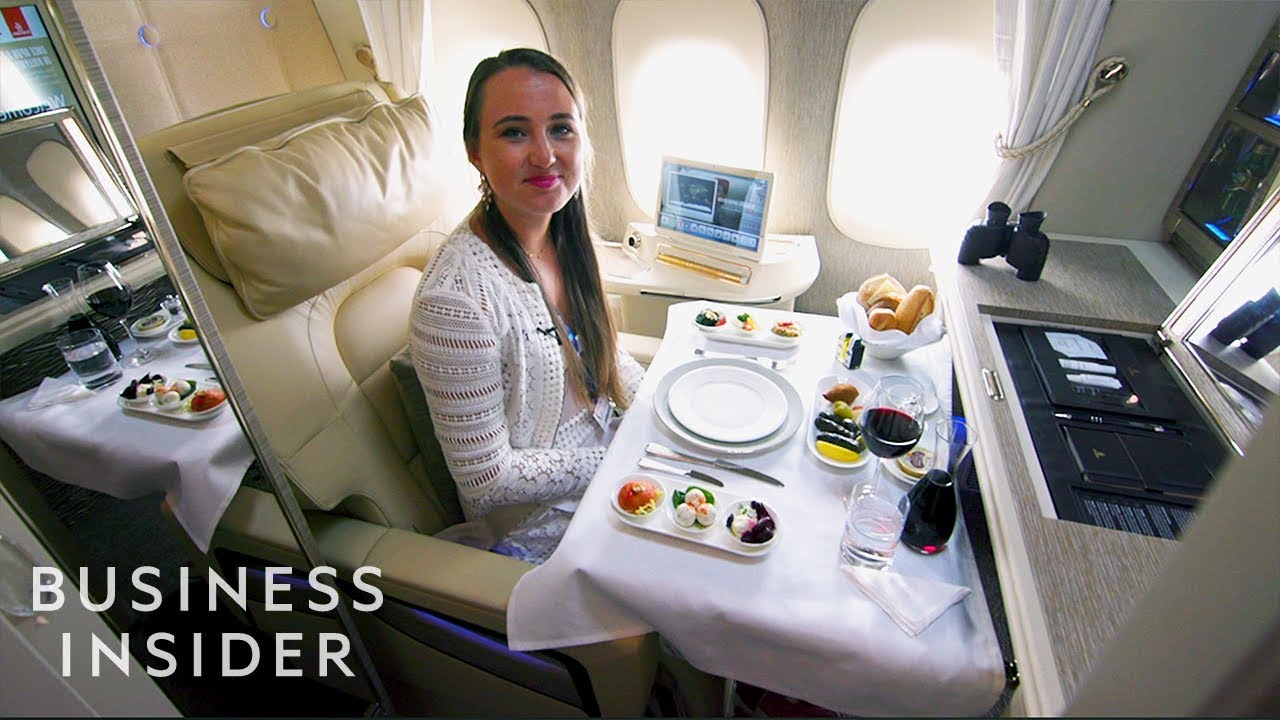In the image, a young woman, appearing to be between 17 and 25 years old, is sitting in a luxurious setting that resembles a first-class airplane cabin. She is seated on a plush, large yellow chair linked to another behind her, forming cozy, booth-like compartments. Her long brown hair cascades down, and she is adorned in a white long-sleeve sweater. Her makeup is meticulous, featuring pink lipstick and eye makeup, enhancing her youthful and sophisticated appearance.

In front of her is a table draped with a white tablecloth, set with an empty white plate nested inside another, reflecting a meticulous arrangement. Flanking the plates are large and small knives, while surrounding them are several trays filled with an array of fine foods, including vegetables, desserts, cookies, and a basket of bread rolls. A wine glass filled with a dark liquid, possibly wine or juice, is also present, suggesting that she might be an entrepreneur or someone of refined taste. A pair of binoculars sits on the table, and a mirror is visible behind her.

In the bottom left corner of the image, "Business Insider" is clearly written in white, indicating the source or context of the photograph. The woman exudes an air of elegance and poise as she looks directly at the camera, capturing a moment of serene luxury.